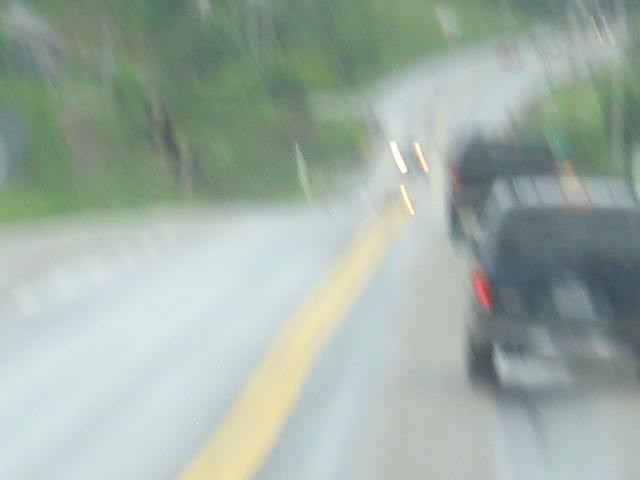A shaky photograph, likely taken from within a moving vehicle on a rainy day, captures the experience of driving through a bustling highway or busy road in a town or city. The wet streets reflect the overcast weather, with raindrops visible on the windshield. The image shows cars traveling in both directions; the bright headlights of oncoming traffic contrast with the red brake lights of vehicles ahead, hinting at an upcoming stoplight or intersection. Flanking the road, lush greenery and trees add a scenic backdrop to the otherwise dreary weather conditions, creating a blend of natural beauty amidst urban commotion.